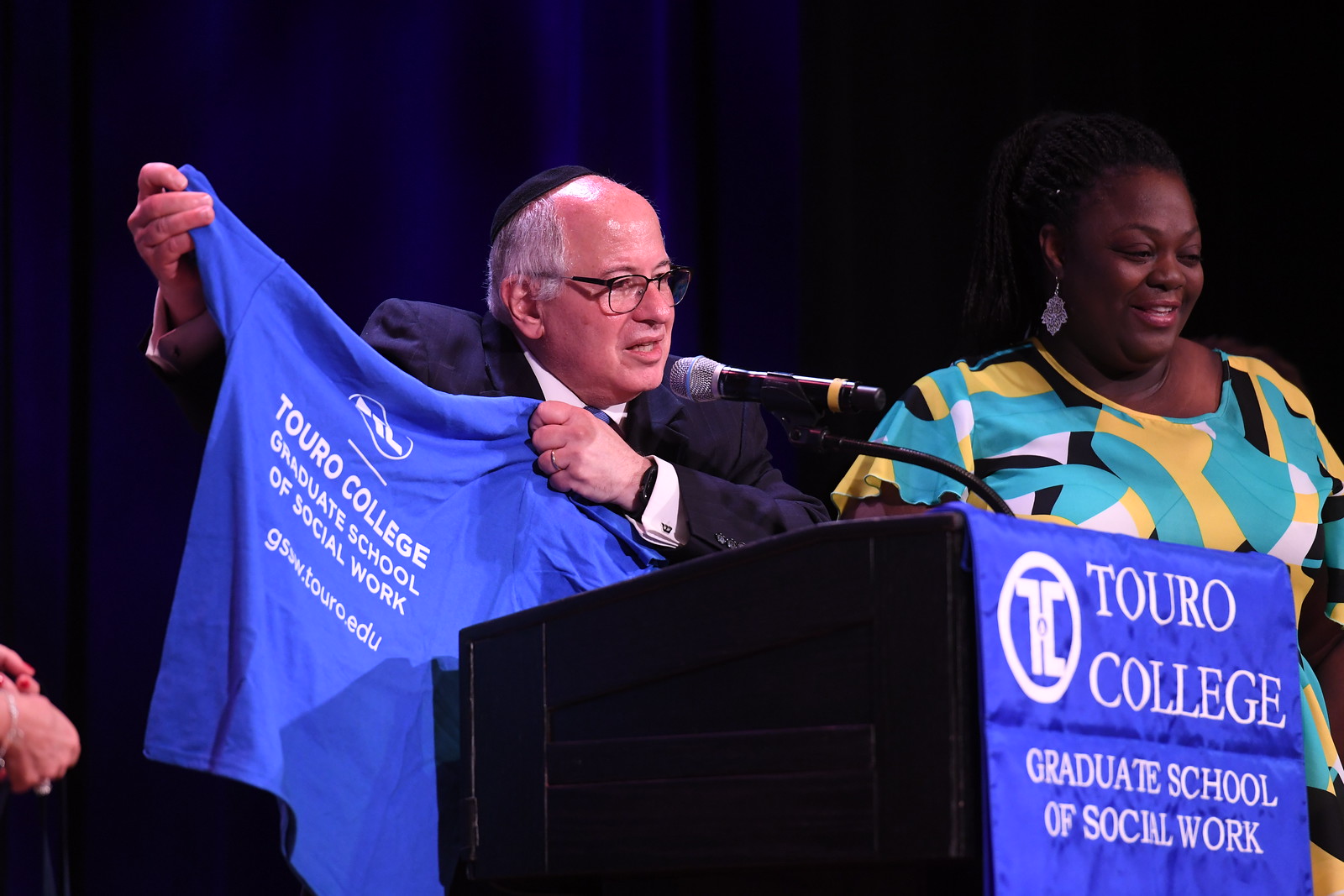In this rectangular photograph, a group of people is gathered on a stage with dark blue curtains in the background. At the center, a gentleman in a dark navy suit, white shirt, blue tie, and glasses is speaking into a microphone at a podium adorned with a blue banner reading "Touro College Graduate School of Social Work" in white letters. He is holding up a matching blue t-shirt with the same white lettering and the college's website beneath it. The man also wears a yarmulke. To his right stands an African-American woman, smiling and wearing a brightly patterned dress in shades of turquoise, yellow, blue, and black, along with dangly earrings. On the left side of the image, only a pair of hands is visible, suggesting the presence of another person just out of frame.